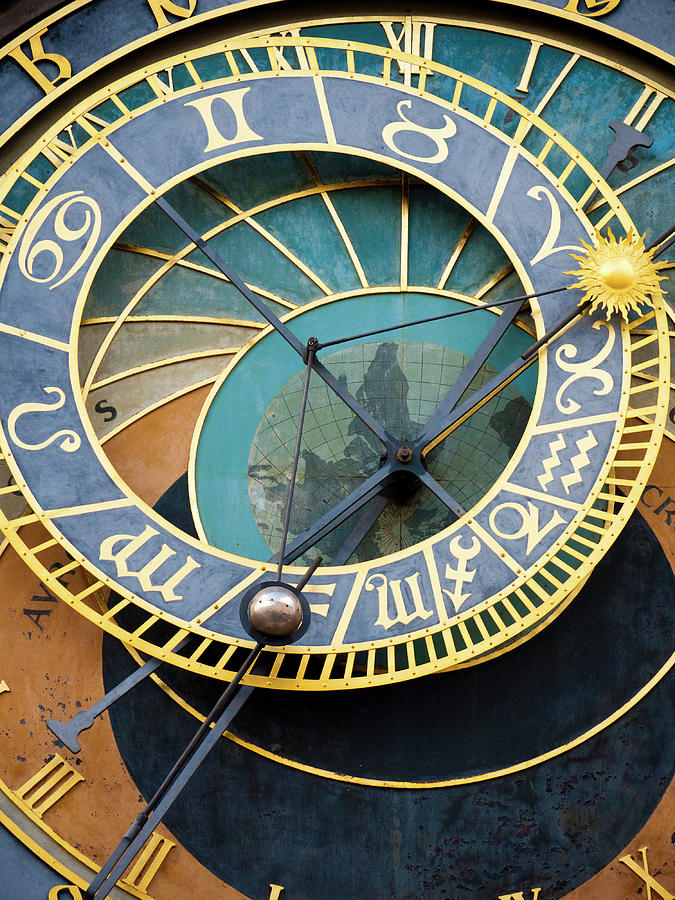The image is a highly detailed, photorealistic depiction of a vintage, astronomical clock. It features a large, intricate main dial adorned with Roman numerals for the times, set against a pale orange and blue background. This main clock face is complemented by an astrological clock floating above it, displaying various zodiac symbols within distinct sections. The clock hands are a striking blue, and there's a prominent golden sun on one end of a hand, mirrored by a silver moon on the lower left. The astrological dial is bordered by a gold railing-like edge, adding to its ornate beauty. Behind the clock faces, a vibrant, colorful globe of the Earth is visible, patterned in blue, orange, and metallic gold. This exquisite piece appears to be a historical clock, possibly from Germany, designed not only to tell the time but also to change with the months and years, and to forecast eclipses.